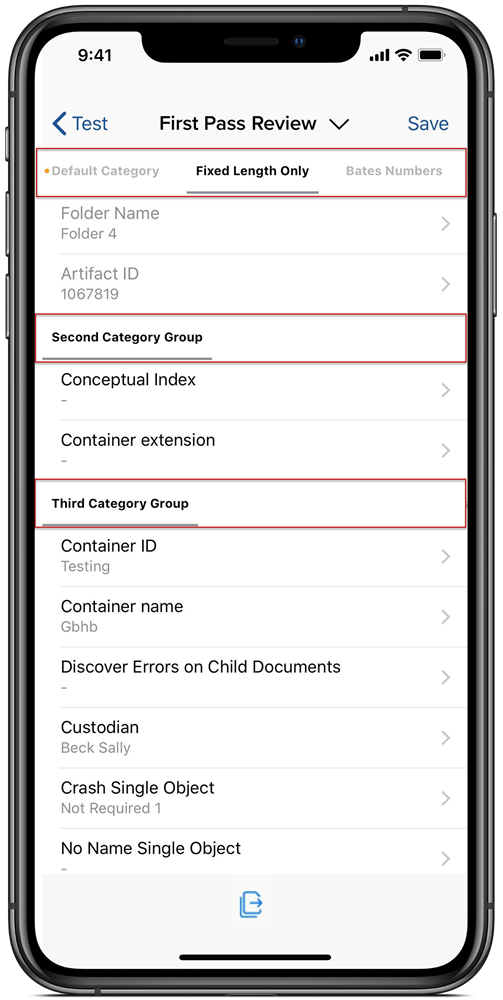A close-up image of an Apple iPhone displaying a coding or software review application. The screen prominently features the heading "First Pass Review" at the top. Below this heading, there are three selectable categories: "Default Category," "Fixed Length Only," and "Bates Numbers." The "Fixed Length Only" option has been selected. Further down, two subcategories are listed: "Second Category Group" and "Third Category Group." The image appears to be focused on showcasing the interface of a coding or software development tool designed for categorizing and reviewing code.